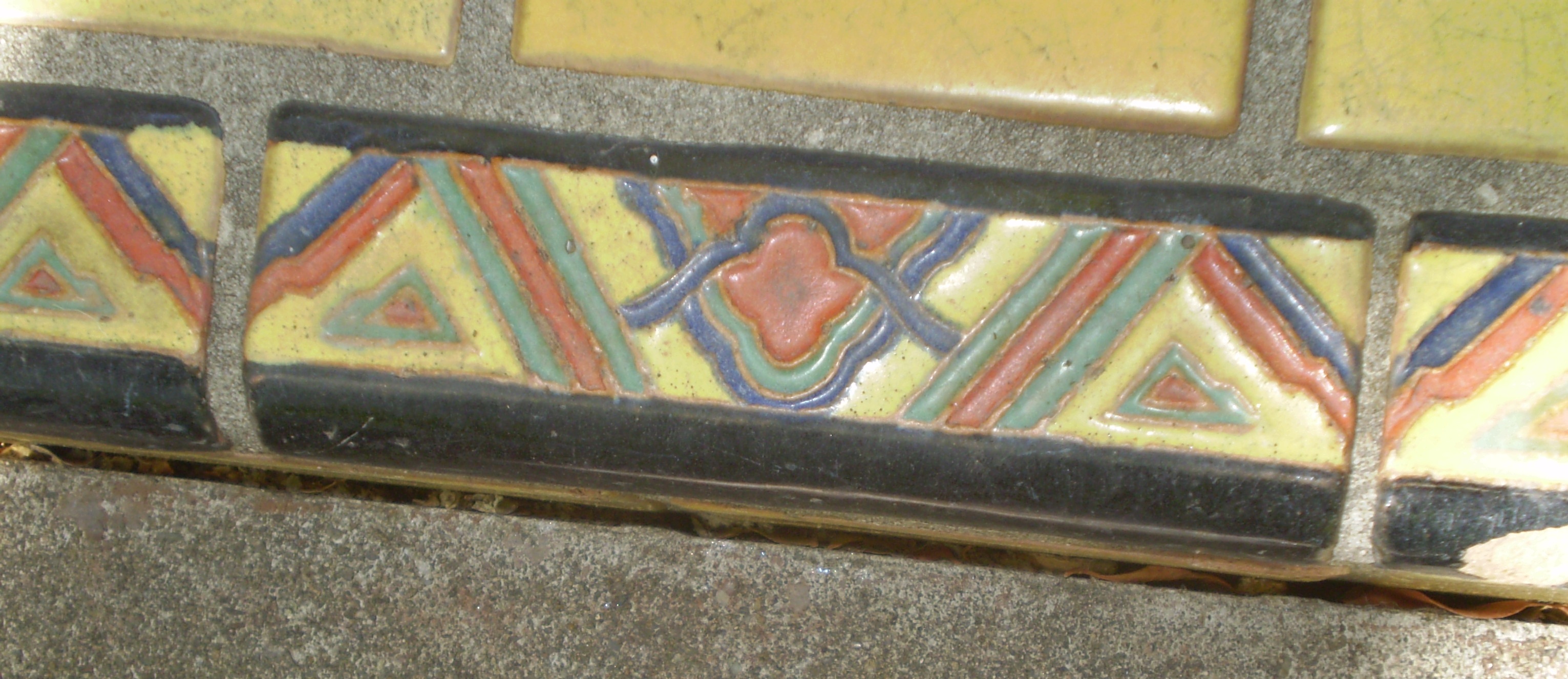The image depicts a detailed and colorful rectangular tile wall, possibly located at the corner of an outdoor counter or in someone's backyard. The wall is constructed from rectangular tiles arranged in a zigzag pattern, with the lines forming the zigzags being of various colors such as blue, red, and green. The tile background is primarily yellow, and the zigzag pattern adds a dynamic, up-and-down visual rhythm. 

There is an element resembling an upside-down triangle cutting through the middle of the rectangle, introducing additional geometric interest. The overall composition is horizontal, featuring a mixture of shapes including triangles and circular forms. These shapes and vibrant colors—yellow, green, blue, and red—create an almost floral pattern.

On the right side, light reflection suggests that the scene could be outdoors, and below the tiles, there is a cement base with a narrow gap that could easily swallow thin items like loose change or a cell phone. Grout fills the spaces between the yellow tiles, adding a clear boundary to each colorful segment and enhancing the meticulous craftsmanship of the tiling work.